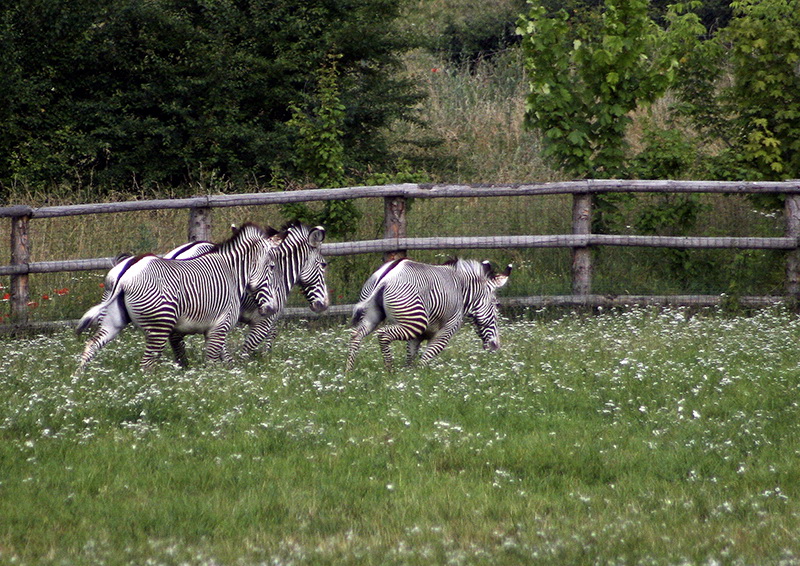This image captures a vibrant zoo exhibit featuring three zebras in full stride across a grassy field dotted with small white wildflowers. The smallest zebra leads the sequence, followed by two slightly larger ones, all exhibiting dynamic motion. The lush greenery extends beyond the wooden fence with metal wiring that encloses their space. Tall, thick grass and dark, dense trees dominate the background, interspersed with various shrubs, some of which appear yellowed, and medium-sized trees sporting lighter green leaves. The scene is bathed in daylight, enhancing the vivid hues of green that contrast with the zebras' striking black and white stripes and the earthy tones of the brown fence.